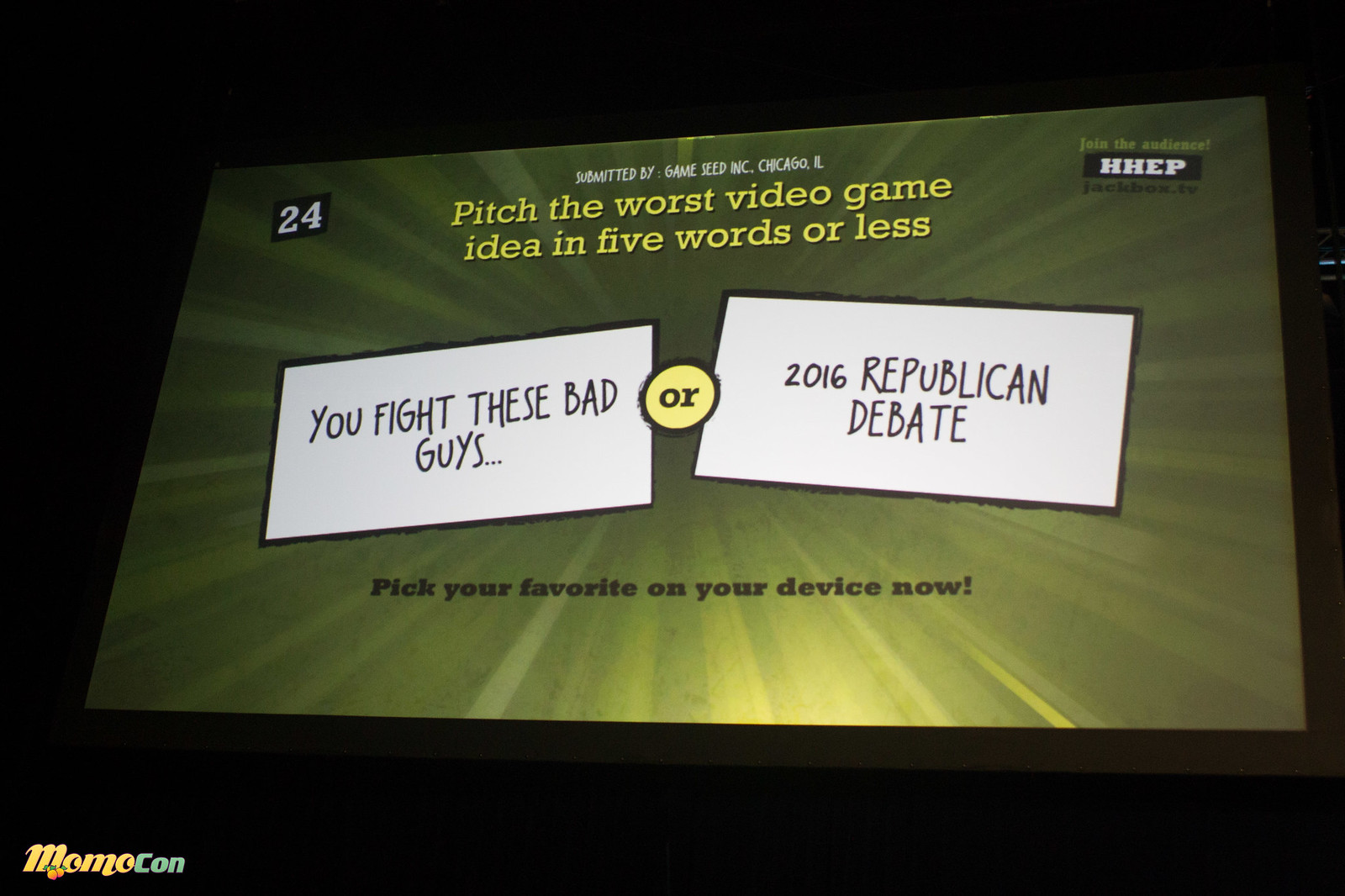The image shows a digital screen with a green, olive-toned background that features rays radiating from the center. Dominating the screen, in bold yellow letters at the top center, is the challenge: "Pitch the worst video game idea in five words or less." Below this prompt, two white rectangles with black borders present the ideas. The left rectangle reads, "you fight these bad guys," while the right one declares, "2016 Republican debate." Between these two rectangles is a yellow circle with the word "or." Towards the bottom, the instruction "pick your favorite on your device now" appears in small black text. In the upper left corner, the number "24" is displayed in white within a black square. Additionally, the very top right corner includes the message "join the audience HHEPjackbox.tv." In the lower left corner of the entire image, not part of the screen, the word "MomoCon" appears in yellow text. The image has an overall faded look, indicating it might be of low quality.